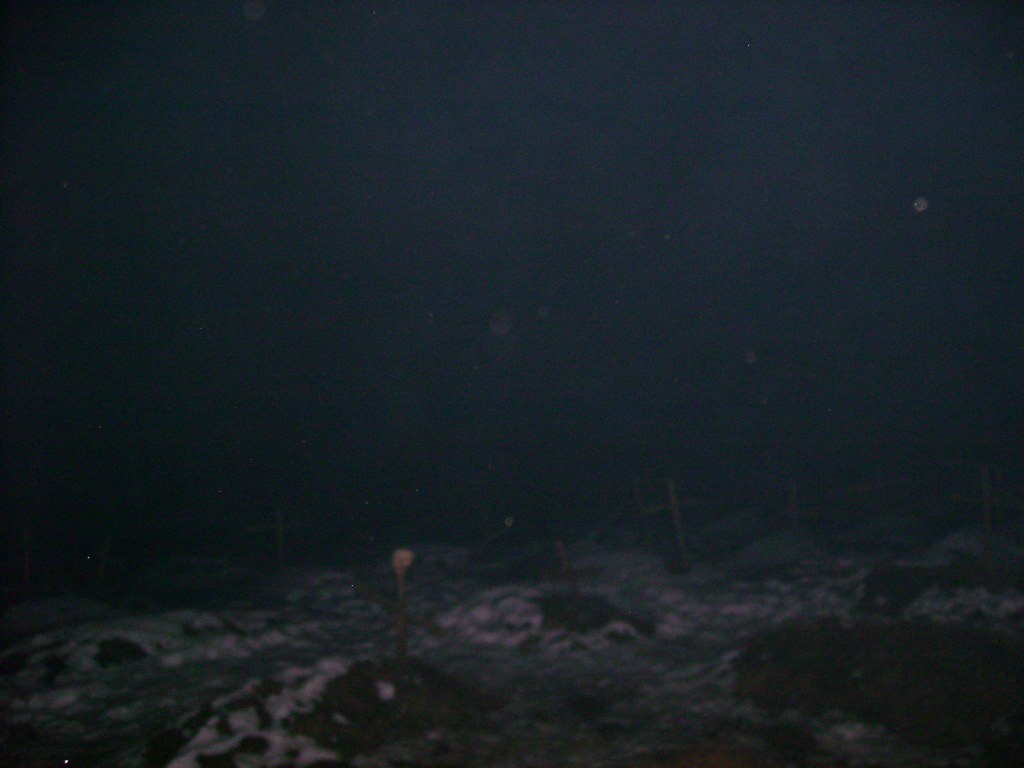In this dimly lit nighttime photograph, the majority of the image is enshrouded in darkness, making it difficult to distinguish specific details, especially in the upper three-quarters of the picture. The dark sky has a faint blue tint with patches of black, and just at the upper right-hand corner, there may be a faint glimpse of the moon. The ground covered in a mixture of light and dark gray hues with patches of white snow reveals a desolate scene. There are piles of snow on what could be a dirt path or a traveled road towards the left. Scattered across the ground, which partially peeks through the snow, are several simple wooden crosses, some leaning slightly forward. One noteworthy structure appears to be without the cross portion, potentially bearing a skull at its top. These elements suggest the area may be a burial ground or cemetery shrouded in heavy shadow, with snow lightly covering the gravesites. The overall graininess and blurriness due to the low lighting conditions contribute to the eerie and somber atmosphere of the photograph.